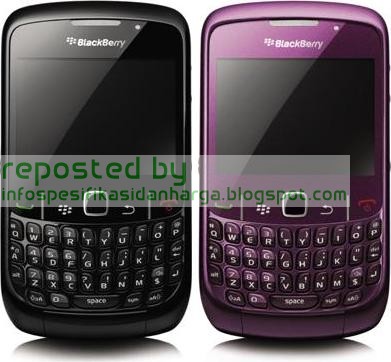This square color photograph features two BlackBerry phones positioned side by side against a solid white background, lending the devices an appearance of floating. Each phone displays the iconic BlackBerry logo, centered at the top in white text with a small logo beside it. The device on the left is black with a matching black keypad, where white letters and numbers are clearly visible. To its right is a purple BlackBerry phone of the same model, featuring a purple keypad with white text. Both phones have large blank screens situated above their keypads. Across the center of the image, there is an imposed horizontal banner in a light white tint with green text that reads, "Reposted by," followed by an indistinct blogspot.com address. The image combines photographic realism with elements of graphic design and typography, adding a slight drop shadow at the bottom of the phones, emphasizing their form and placement.